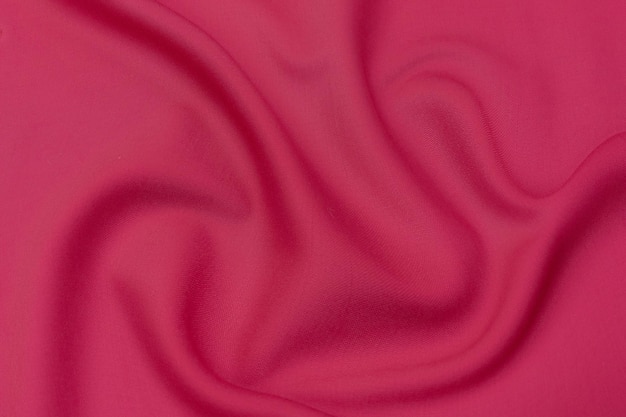A vibrant, neon pink cloth fills the frame of this color image, showcasing a dynamic array of folds and gathers. The fabric's texture is beautifully highlighted, with smooth, flowing curves and intricately bunched sections that create a mesmerizing pattern. Delicate shading along the edges of the cloth enhances the depth and dimension, drawing the viewer's eye towards the center of the composition, where all curves converge. This striking image captures the intricate details of the cloth's surface, emphasizing the interplay between light and shadow.